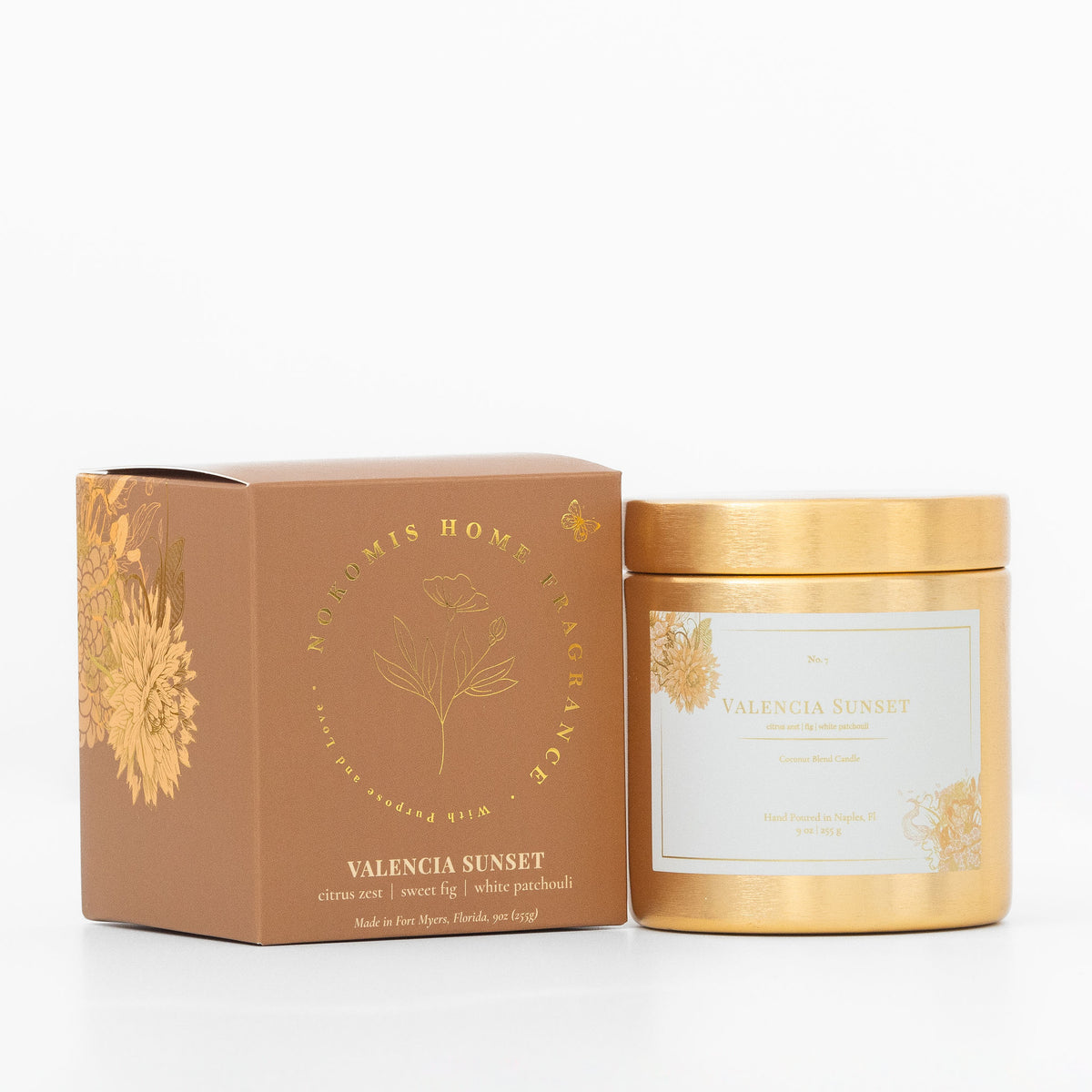In a professional photograph, a beautifully presented scented candle is showcased, featuring a distinctive fragrance called "Valencia Sunset." The candle comes in an elegant jar with a shiny golden hue that complements its label, which is white with matching gold font. The jar sits beside its packaging on a white table, accentuating the product's refined aesthetic. The box is a square, neutral-colored container adorned with gold lettering, including the scent notes: Citrus Zest, Sweet Fig, and White Patchouli. Both the candle and the box are part of the Nokomis home fragrance line, made in Fort Myers, Florida. The box also features a small golden butterfly and floral illustrations, adding to the sophisticated presentation. The overall setup effectively highlights both the candle and its stylish packaging in a white-background setting.